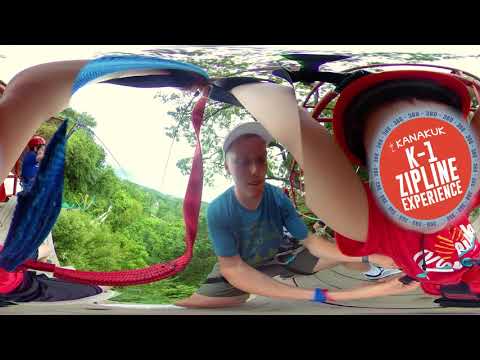In this vibrant and slightly distorted daytime photograph taken in a lush forest setting, a central figure, a man clad in a turquoise-blue shirt and a white hat, is securing a young boy for a zipline ride. The boy, dressed in a magenta-pink shirt and attached to a red or purple strap, stands eagerly to the right, poised for the adventure. Both figures are central to the composition, complemented by a backdrop of abundant greenery with bright green leaves. On the right side of the image, partially superimposed over the boy’s face, is a circular advertisement featuring the text "Kanakook K1 Zipline Experience" in a red circle, further anchoring the thrilling context of the scene.